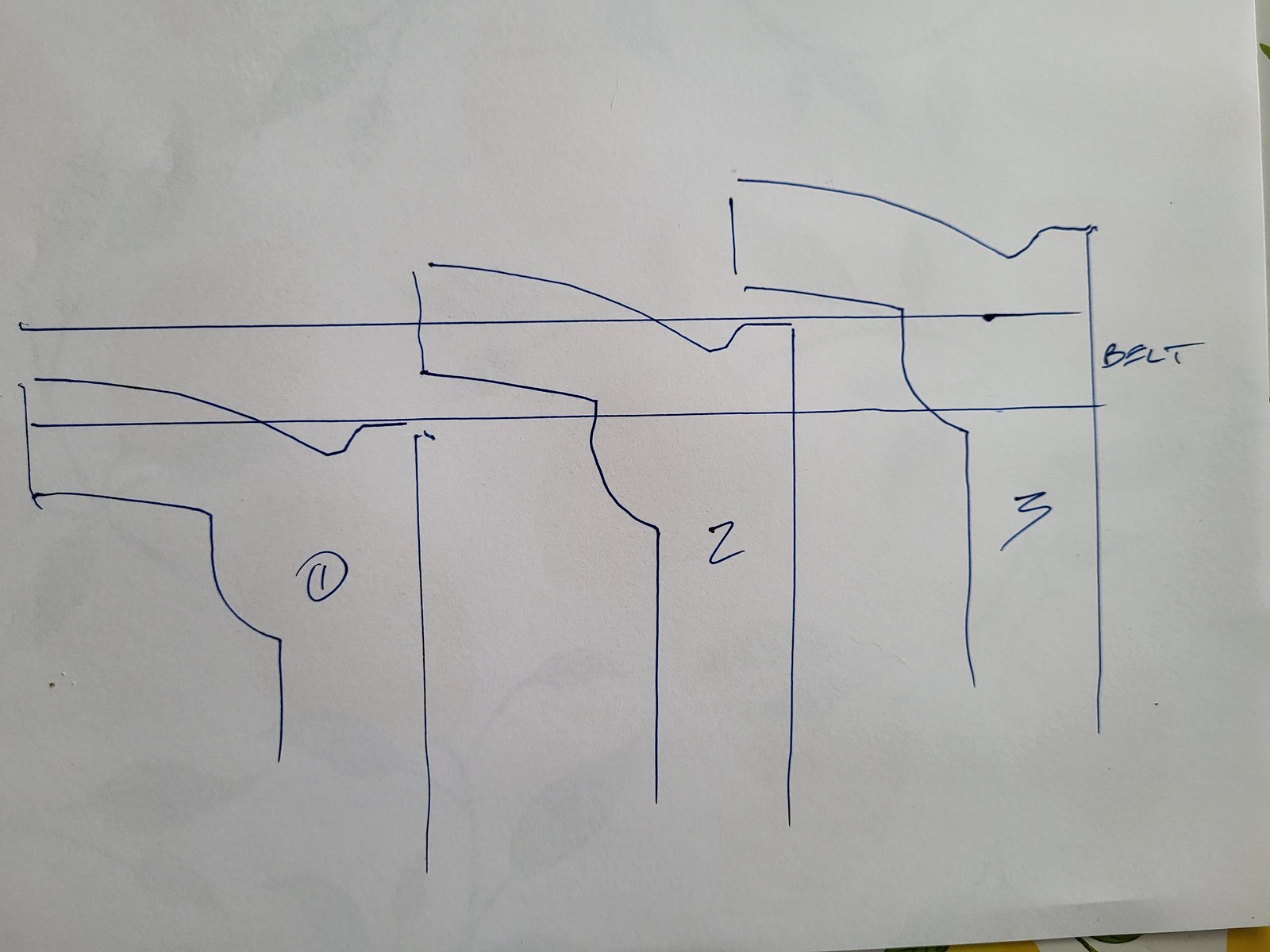This image depicts a clear white piece of paper with blue ink drawings and handwriting. Central to the composition is a long rectangle, labeled "belt" in distinctly masculine handwriting. Alongside the rectangle, there are three line art drawings of guns. Each gun is labeled with a number; on the far left, "1" is circled, the middle gun is labeled "2" but not circled, and the one on the far right is labeled "3," also without a circle. Notably, the ink has bled slightly near the end of the rectangle. The background is minimal, revealing just a tiny sliver of the surface the paper rests on, making it unclear if it is a table or another platform.